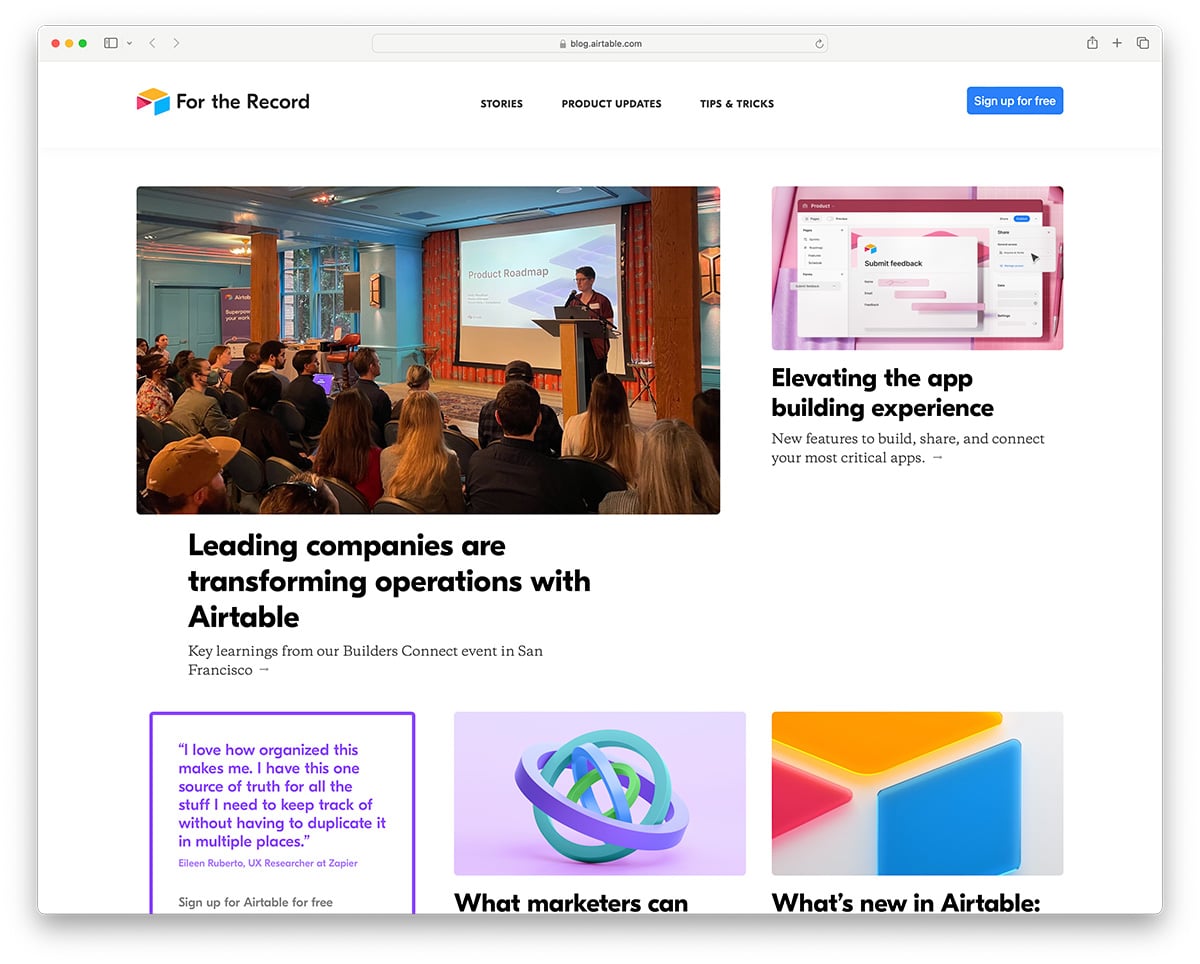This appears to be a captured screenshot of a website. 

At the top, the image features a gray bar with several navigation elements: a trio of dots in red, gold, and green on the left, and a series of gray icons including a square, a back arrow, and a forward arrow. Also present is a white address bar containing the web address "blog.something.com" accompanied by a black padlock icon, indicating a secure connection. A refresh button is seen on the right side of the address bar. Further to the right are icons for a document with an upward arrow, a plus sign, and another document icon.

Beneath the navigation bar, the main content area starts with a colorful section featuring shades of pink, orange, and blue. It has a black header stating "For the Record" followed by subheadings "Stories, Product Updates, Tips, and Tricks." Beside it, a blue and white box prompts users to "Sign Up for Free."

In the middle of the page, there is an image depicting a person speaking at a podium in a conference room filled with men and women seated. A noticeable projection screen is set up in the room. Below this image, a text block reads in black, "Leading companies are transforming operations with Airtable. Key learnings from our Builders Connect event in San Francisco." Following this is a testimonial in purple, "I love how organized this makes me. I have this one source of truth for all the stuff I need to keep track of without having to duplicate it in multiple places," alongside the person's name. Below, a CTA reads "Sign up for Airtable for free."

At the bottom, a purple background features a series of icons in purple, green, and teal, with partially visible text, "What Marketers Can."

On the right, another segment contains geometric shapes in pink, gold, and blue, alongside a black header, "What's New in Airtable."

The topmost section highlights another series of images in pink, white, black, and blue color schemes, headlined in black text, "Elevate an App Building Experience, New Features to Build, Share, and Connect Your Most Critical Apps."

Overall, the screenshot captures a detailed snapshot of the webpage including its navigation elements, vibrant segments, promotional content, and calls-to-action.